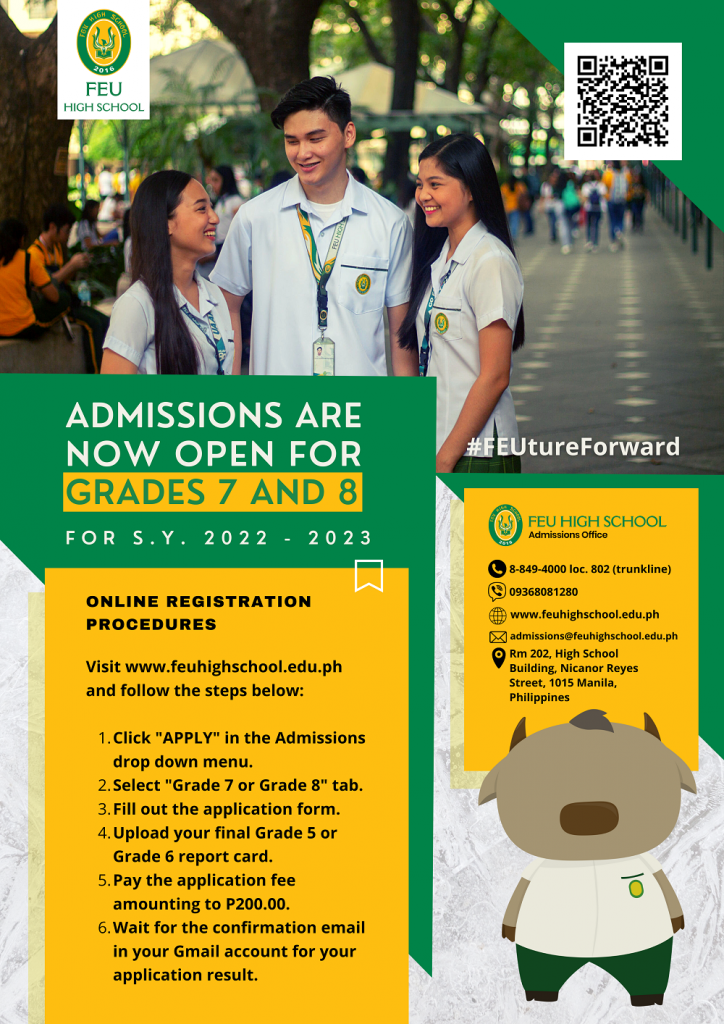In the image, a young man is flanked by two women, both wearing light blue shirts. They stand on a gray ground. To the right of them is a scan code, with a green triangle section just above it. On the left side, trees provide a natural backdrop. 

In the center, there's a square featuring a green circle and an orange circle inside it, with the text "FEU High School" displayed underneath. Below this, in green boxes with white font, it reads, “Admissions are now open,” followed by an orange box with green lettering indicating grades seven and eight. Further down, in white text, it states "for s.y. 2022-2023."

Below this information, highlighted in an orange background with black font, the text instructs: "Online registration procedures, visit www.feuhighschool.edu.ph and follow the steps below." 
1. Click 'Apply' in the admissions drop-down menu.
2. Select the Grade 7 or 8 tab.
3. Fill out the application form.
4. Upload your final Grade 5 or Grade 6 report card.
5. Pay the application fee amounting to Php 200.
6. Wait for the confirmation email in your Gmail account for your application results.

On the right side, in white font, it reads "FEU Tier Forward" next to a green triangle followed by an orange square. The green lettering continues with "FEU High School" and in black, "Administration Office," followed by a list of phone numbers, physical addresses, and email addresses for contact.

Additionally, there is a small, gray creature with a brown nose and brown horns atop its head, dressed in a white shirt and green pants, adding a friendly and whimsical touch to the promotional content.